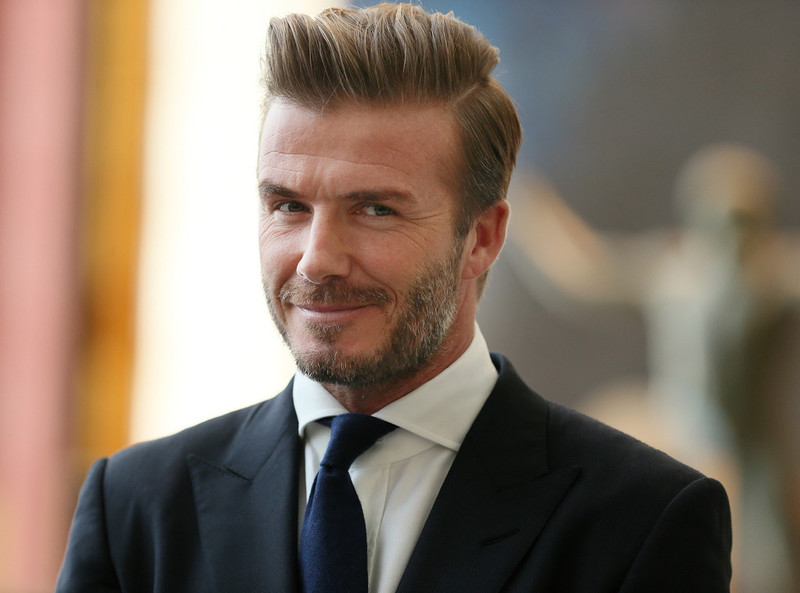In this close-up image, we see the renowned soccer star David Beckham in what appears to be his early to mid-40s, exuding an air of sophistication and charm. Beckham, who might be attending a charity event or similar significant occasion, is attired in a dark navy blue suit paired with a white dress shirt and a dark tie. His meticulously styled hair, complete with a slight quiff, and his well-groomed beard, tinged with white around the edges, add to his distinguished appearance.

Beckham's captivating grayish-blue eyes and his subtle smirk, coupled with a side-eye glance, convey a sense of contentment and confidence. Despite the blurry background, which features bands of color including pink, yellowish-orange, white, and a vague grayish figure that might be a sculpture or painting, the focus remains squarely on Beckham. The photograph highlights his attractive features, slight wrinkles around his eyes, and an overall happy demeanor, making it an excellent portrait that could be ideal for a book cover or as a professional headshot.